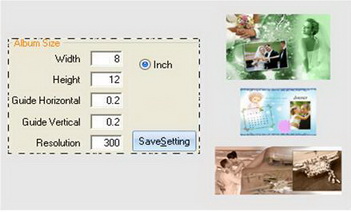The image displays a light gray computer screen showing a web interface for creating a photo album. On the right-hand side are three sets of digital images: the first set has a greenish hue featuring a wedding scene with a man, woman, and officiant, and hands visible in the top left corner; the second set has a blue background with a woman on the left and a couple on the right hugging, along with another couple in a black-and-white picture presumably near the ocean; the third set is sepia-toned or black and white featuring more wedding-related imagery. On the left side of the screen, within a tan box with a dashed border labeled "Album Size," there are input fields for width (8 inches), height (12 inches), horizontal guide (0.2), vertical guide (0.2), and resolution (300 dpi). Below these fields, there's an option to choose the unit (inches selected here) and a "Save Setting" button located at the bottom right of the box.